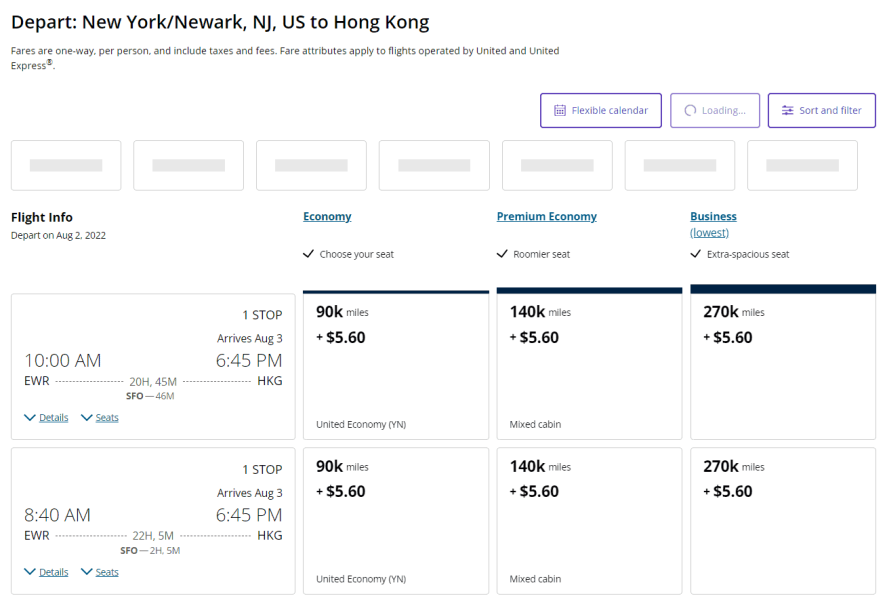In this image, we see a detailed flight information screenshot prominently displayed in the upper left-hand corner. The information outlines a journey departing from New York/Newark, New Jersey, U.S. to Hong Kong, specifying that fares are one-way per person and inclusive of taxes and fees. It notes that fare attributes apply to flights operated by United and United Express.

The interface provides options to use a Flexible Calendar, with features for Loading, Sorting, and Filtering the available flights. The specific flight information for a departure on August 2nd, 2022, is shown, detailing options across different classes of service: Economy, Premium Economy, and Business. Economy allows passengers to choose their seats, Premium Economy offers roomier seating, and Business class, described as "Extra Spacious Seat," is the lowest pricing tier mentioned.

The highlighted flight departs at 10 a.m. from EWR (Newark Liberty International Airport), with a total duration of 20 hours and 45 minutes, including one stop, arriving in Hong Kong at 6:45 p.m. on August 3rd. Pricing details in the left section indicate mileage costs: Economy at 90,000 miles plus $5.60, an intermediate tier at 140,000 miles plus $5.60, and the highest tier at 270,000 miles plus $5.60. Another flight option listed departs at 8:40 a.m., has a duration of 22 hours and 5 minutes, and also arrives at 6:45 p.m. in Hong Kong.